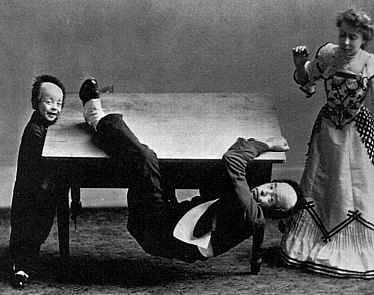In this black and white photograph, three individuals are captured in what appears to be a comedic scene set against a plain dark gray wall. Central to the image is a wooden table that is being tilted forward by a small boy on the left, who looks around five or six years old. The boy, who appears to have short hair and is dressed in a black suit with black shoes, smiles directly at the camera while leaning his head against the table. 

Hanging precariously from the table is a man dressed in a black jacket or shirt and black pants, with his left arm and leg resting atop the table while the rest of his body dangles underneath, close to the ground. The scene gives the impression that the man is about to fall due to the boy's playful antics. 

On the right side of the photograph stands a woman in a long, intricately patterned dress, featuring artistic diagonal lines and crisscross patterns up to the blouse area. Her hair is curly and pinned up stylishly, evoking an old Victorian look. She gazes downward at the man with a look of concern, clearly surprised by the unfolding scenario. The overall composition suggests a playful, lighthearted moment captured in time.